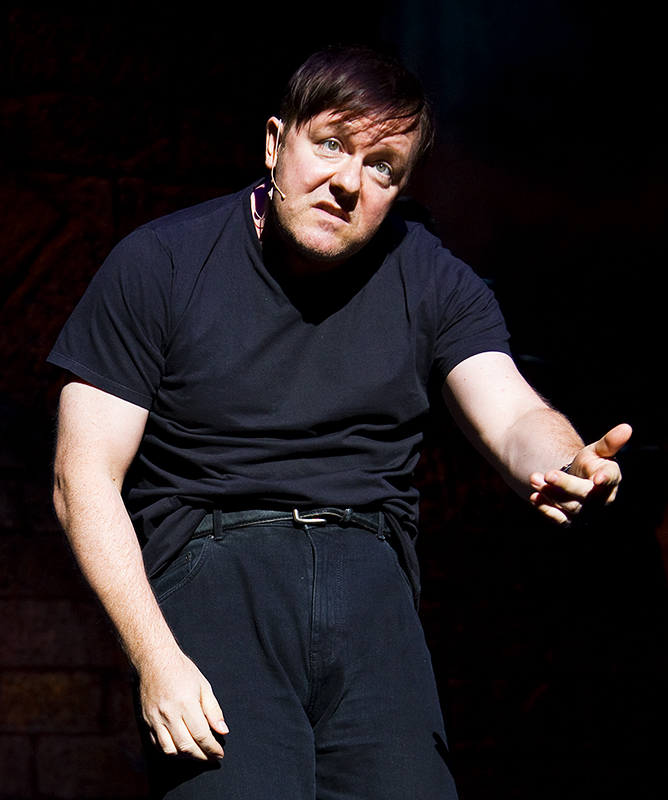In the image, set against a total black background, a performer dressed entirely in black is captured in a moment of dynamic expression. He is clad in a black t-shirt and black pants, accentuated by a black belt with a brass buckle, and part of his shirt is slightly hitched up over the belt. The performer is leaning forward with intense focus, evidenced by the way his dark brunette hair falls and his gaze shifts slightly to the left. His mouth is open as if in the midst of explaining a point, amplified by a performance microphone that sits snugly near his cheek. His left arm, seen on the right side of the photo, extends outward with fingers slightly bent, emphasizing his gesticulations. His right arm, relaxed and slightly bent, rests down by his upper thigh. The bare arm and overall body language convey energy and engagement, drawing viewers into his performance.